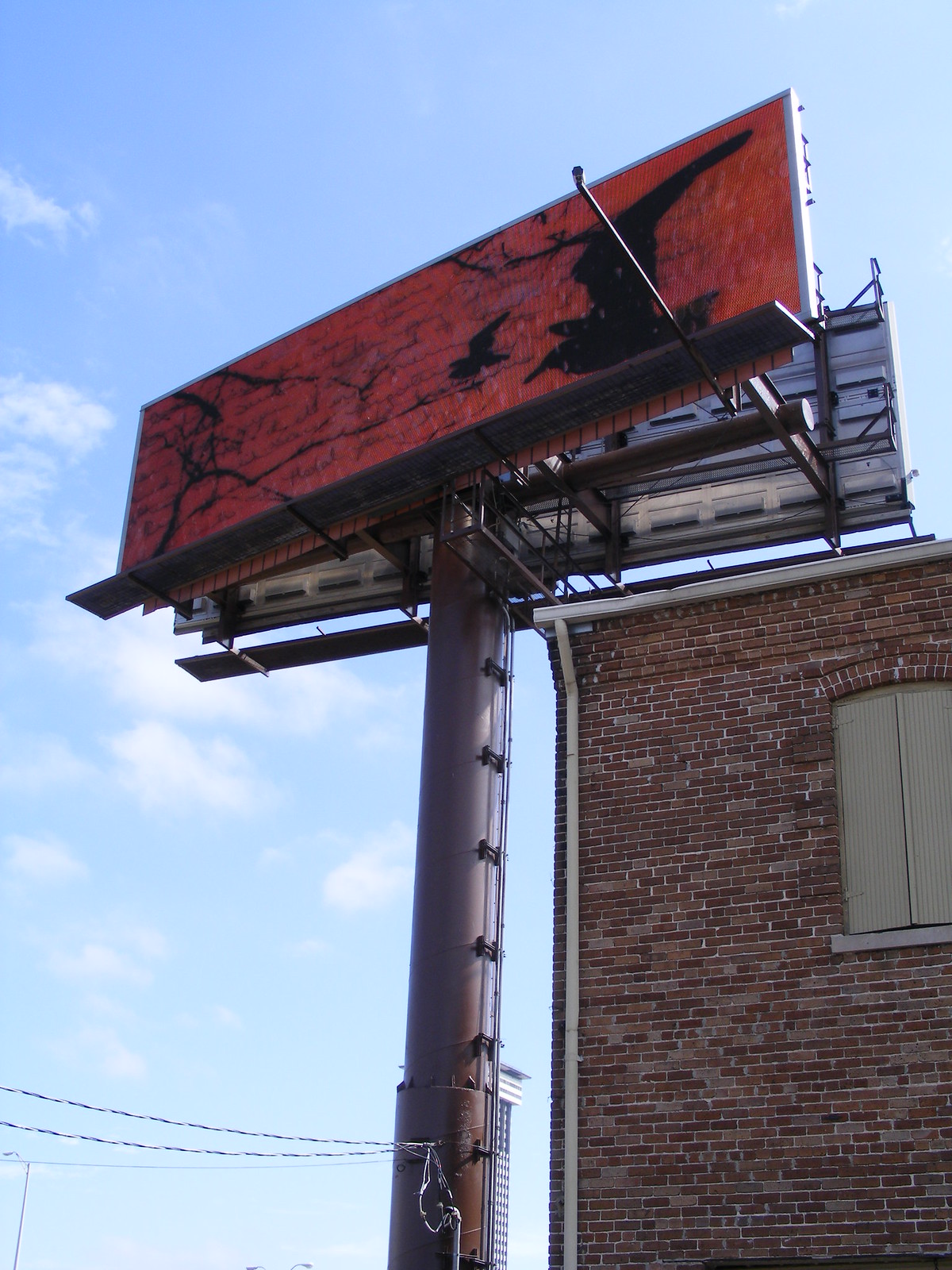The photograph features a compelling optical illusion where a billboard appears to be mounted directly onto a nearby building due to the alignment and perspective. The foreground showcases a red and orange brick building, complete with a gutter system and an elongated downspout. At the apex of this building, there is a solitary window, securely closed with solid shutters. In the background, a tall metal pole supports two billboards. The billboard that faces towards the viewer mimics the cracked and broken appearance of red bricks, blending seamlessly with the building's facade and creating the illusion of damage. The reversed billboard faces away from the camera, adding depth to the scene.